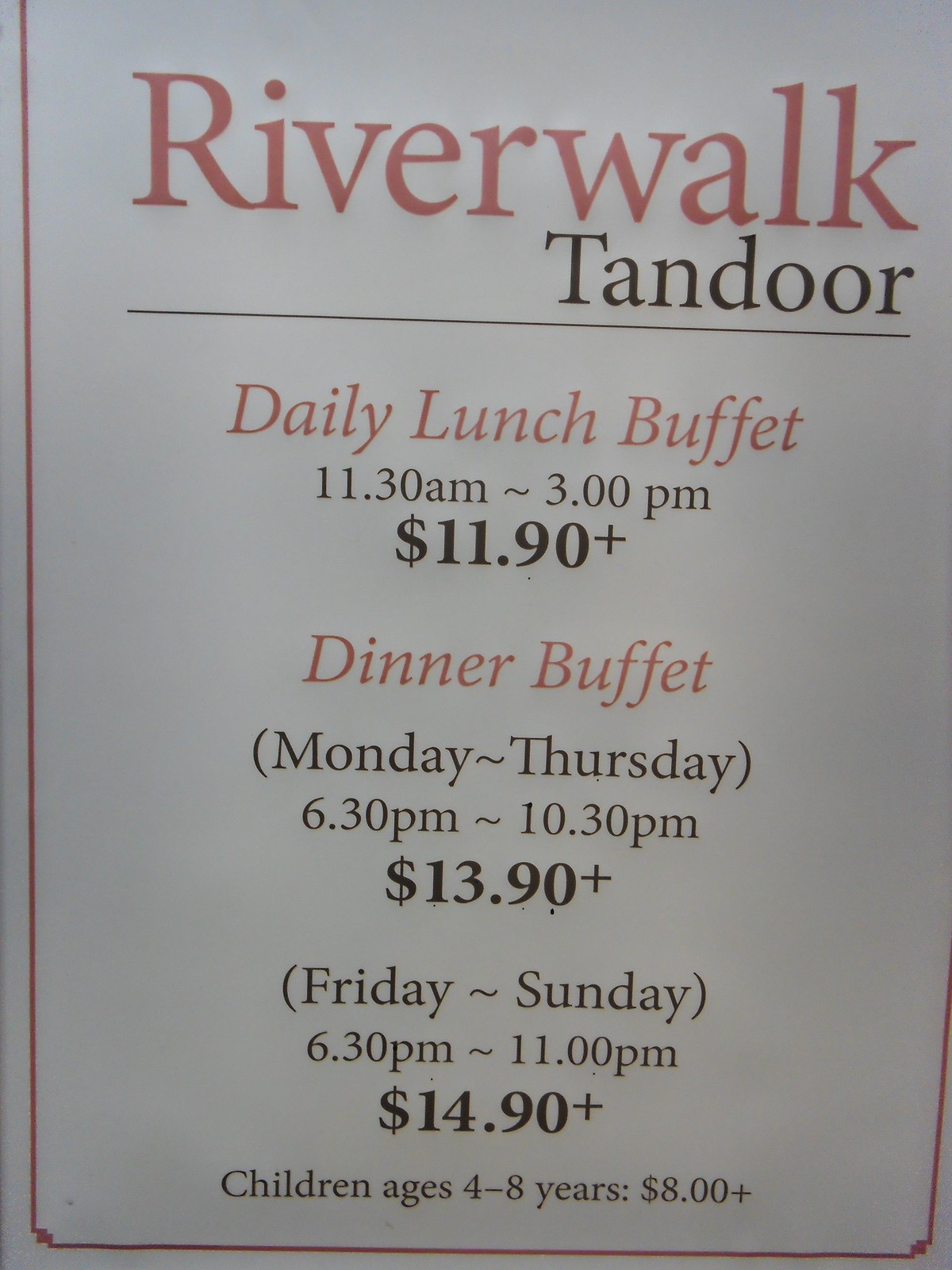The image depicts a restaurant menu on white paper with a light red border. The title "Riverwalk" appears at the top in light red text, with "Tandor" positioned on a second line, justified to the right, in a smaller black font. A thin horizontal black line separates the title from the menu sections below. The menu highlights two main offerings: "Daily Lunch Buffet," listed in red italics, available from 11:30 AM to 3:00 PM for $11.90. The "Dinner Buffet" section, also in red italics, is divided into two subsections. From Monday to Thursday, dinner is served from 6:30 PM to 10:30 PM for $13.90, while Friday to Sunday, it extends until 11:00 PM for $14.90. Children's pricing for ages 4 to 8 is noted as $8+, with all prices in bold font for emphasis.